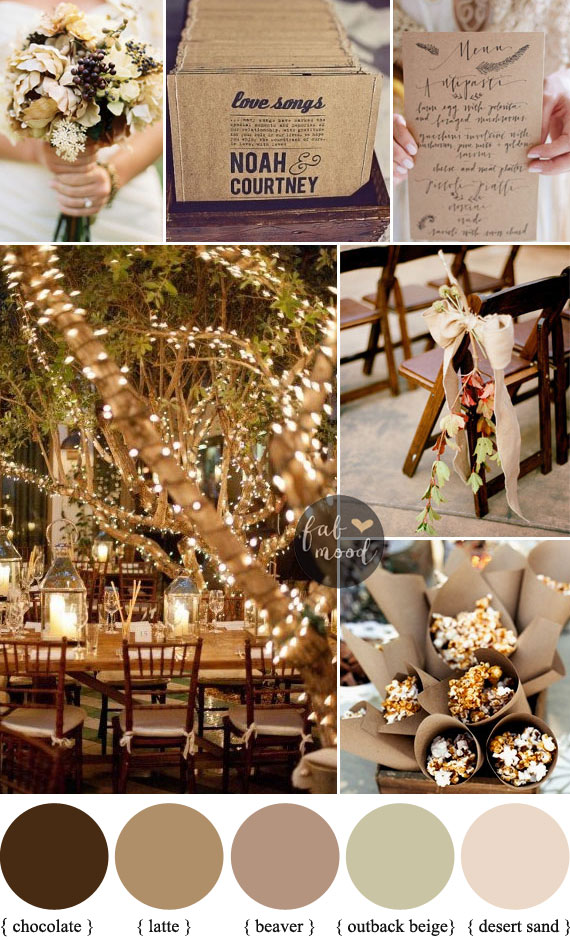The image presents a meticulously curated wedding design theme, likely resembling a Pinterest collage, featuring an array of photographs and graphic elements. At the top, three vertical photos span the width of the collage. The first image captures a bride in a white dress holding a bouquet of dried cream-colored flowers accented with purple berries. The second photo, centered, showcases a rustic setup with pieces of beige paper stacked on a wooden block, displaying the names "Noah and Courtney" under the phrase "love songs." The third picture portrays a bride holding an invitation card.

Below these, the collage transitions into an outdoor wedding scene illuminated by LED lights, with a beautifully decorated table set among trees. Adjacent to this, there are images of chairs adorned with bows and flowers, and multiple floral bouquets crafted from seemingly paper-like materials. The information at the bottom provides a color palette consisting of five shades: Chocolate, Latte, Beaver, Alpaca Beige, and Desert Sand. The central circle features the brand "Fab Mood," emphasizing the cohesive, aesthetic appeal of the wedding theme.